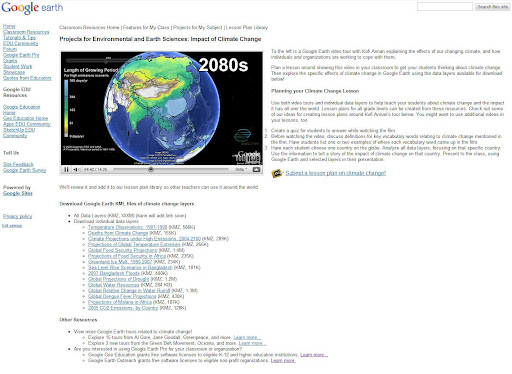This screen capture from the Google Earth website features an interactive web layout. Dominating the upper left corner is the "Google Earth" logo. Adjacent to it, in the upper right corner, a prominent white search bar is positioned beside a distinct gray search button. The left-hand side hosts a vertically arranged sidebar filled with numerous blue hyperlinked texts, each potentially leading to different sections or external pages.

The central area of the webpage is dense with small, black text that is difficult to discern. Among the text, a significant visual element stands out: an embedded image or video player displaying a globe. The visible portion of the globe highlights Asia, prominently showing China, India, Russia, and parts of the Middle East. Overlaying this visual in the upper right-hand corner is white text that reads "2080s," indicating a future-oriented theme or data visualization.